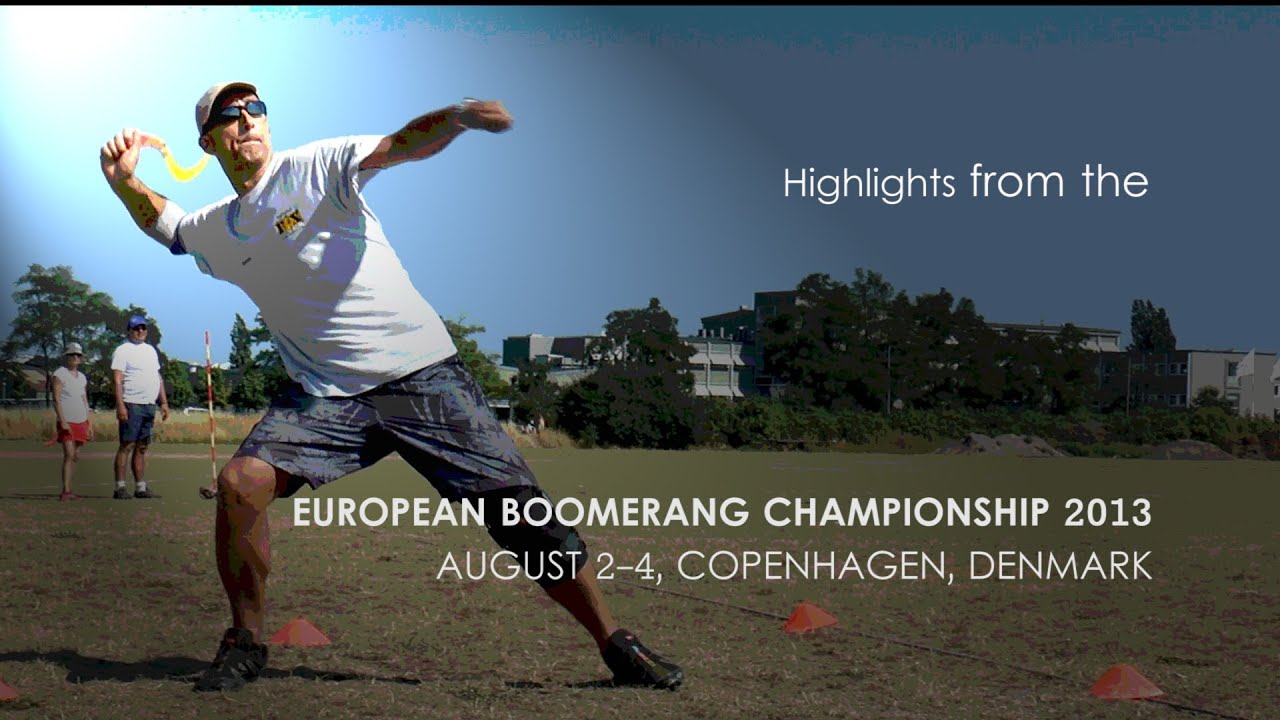The image is a horizontal rectangular promotional banner for the European Boomerang Championship 2013, held from August 2-4 in Copenhagen, Denmark. It features a Caucasian man standing on a grassy field, seemingly about to throw a boomerang. He is dressed in a white t-shirt, Hawaiian-style shorts or possibly khaki shorts, black athletic shoes, a baseball-type hat, and black sunglasses. His posture is dynamic, with his right arm extended upward holding the boomerang, and his left arm stretched out for balance. His right leg is bent at the knee supporting his weight, while his left leg is extended forward. The background showcases a grassy field extending to a grove of trees and buildings on the right. On the left side, two figures, possibly a man and a woman, are watching the action, with some poles and cones visible in the vicinity. The upper right corner features white text reading, "Highlights from the European Boomerang Championship 2013," with further details about the event's date and location in the lower-center part of the image.